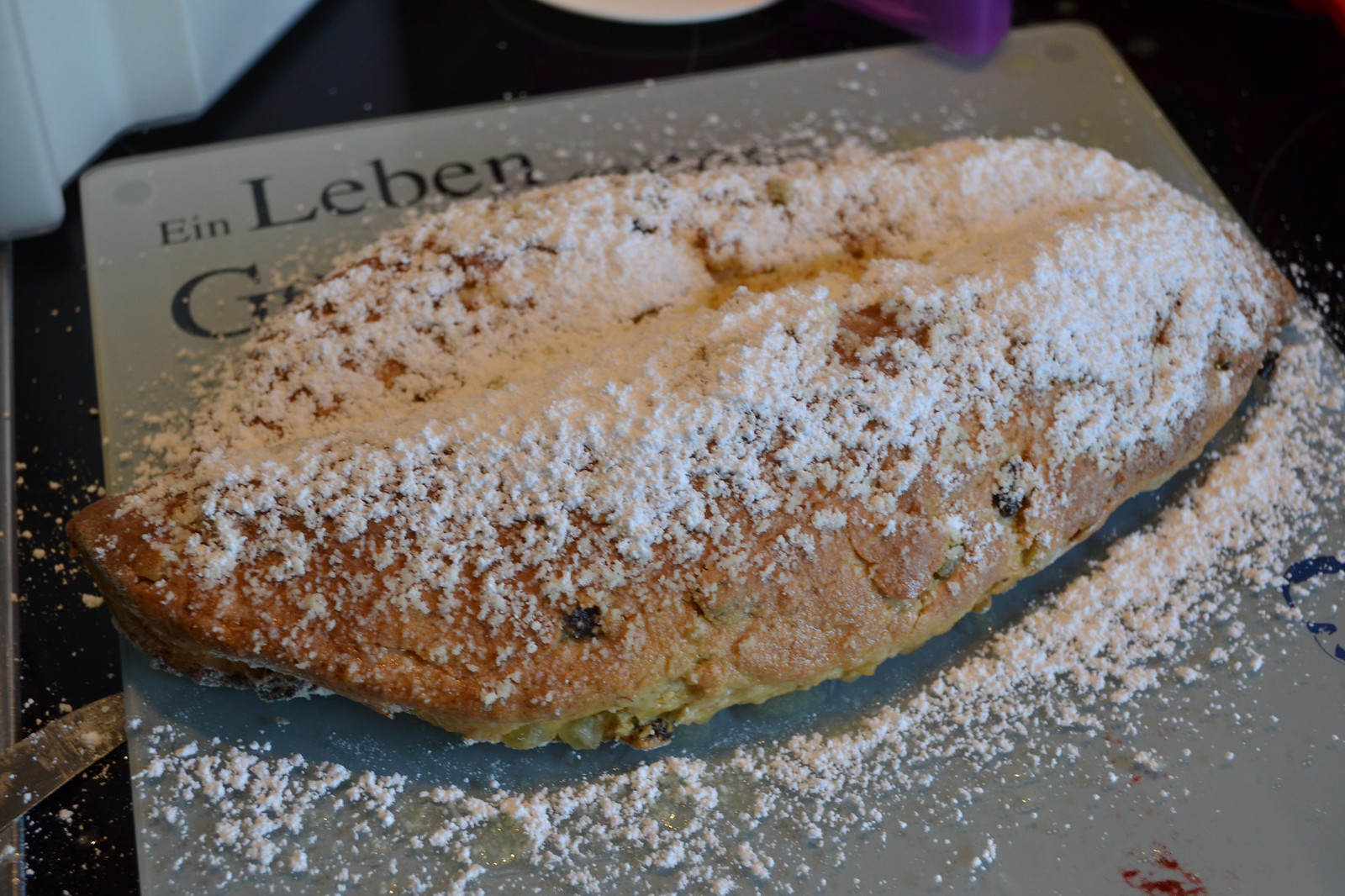In this detailed image, we see a rustic dessert resembling a large loaf of bread or possibly a fruitcake, generously dusted with powdered sugar that covers much of the surface, but still reveals the brownish-tan hue of the dessert itself. The dessert takes on an oval shape and is crafted to look like it has been folded over, similar to an empanada or a pie, with a slight decorative lacy pattern protruding from the front. It lies on a black tablecloth which has crumbs scattered around, indicating it might have been recently sliced or prepared for serving.

The dessert is placed on a cutting board that features the text "Ein Lieben" at the top left corner, with "Lieben" written prominently in larger black letters. Part of a letter "G" is visible, but obscured by the dessert. Near the bottom left corner of the cutting board, the blade of a knife peeks into the frame. The presence of a purple object at the top of the image adds a splash of color, though its purpose is unclear. Additionally, there appear to be a few paint smudges or decorative elements on the cutting board, adding to the overall rustic and homey presentation.

The crumbs and possibly some raisins peeking out from the bottom imply a rich texture, potentially hinting at a raisin bread, although the lack of slices makes the internal composition a mystery. Amid the powdered sugar, there might be small fruits, like grapes, adding to the festive appearance. This image conjures the delightful anticipation of a sweet, hearty treat ready to be enjoyed.